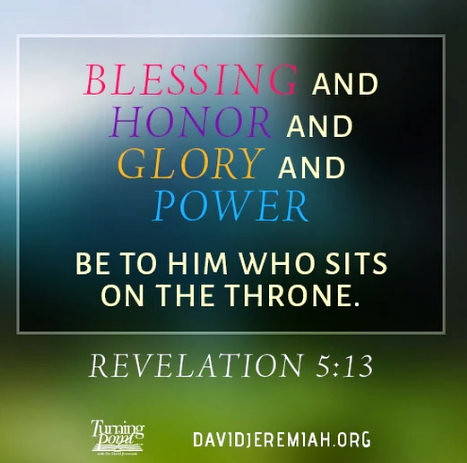The image is a poster with a dreamy, surreal background transitioning from dark blues and blacks at the top to green at the bottom, evoking a hazy, ethereal atmosphere. In the upper left-hand corner, there's a white border surrounding a rectangular frame with text inside. The text reads "BLESSING" in red, "HONOR" in purple, "GLORY" in yellow, and "POWER" in blue, all in capital letters. Below these words, it says "be to him who sits on the throne." in white print. Further down, a citation reads "Revelation 5:13" in white text. The background appears to depict a blurred landscape, possibly a mountainside transitioning into the sky, with colors shifting from greens to blues and whites. At the bottom of the poster, there's a logo for Turning Point on the left. On the right side, the text "davidjeremiah.org" is also in white.